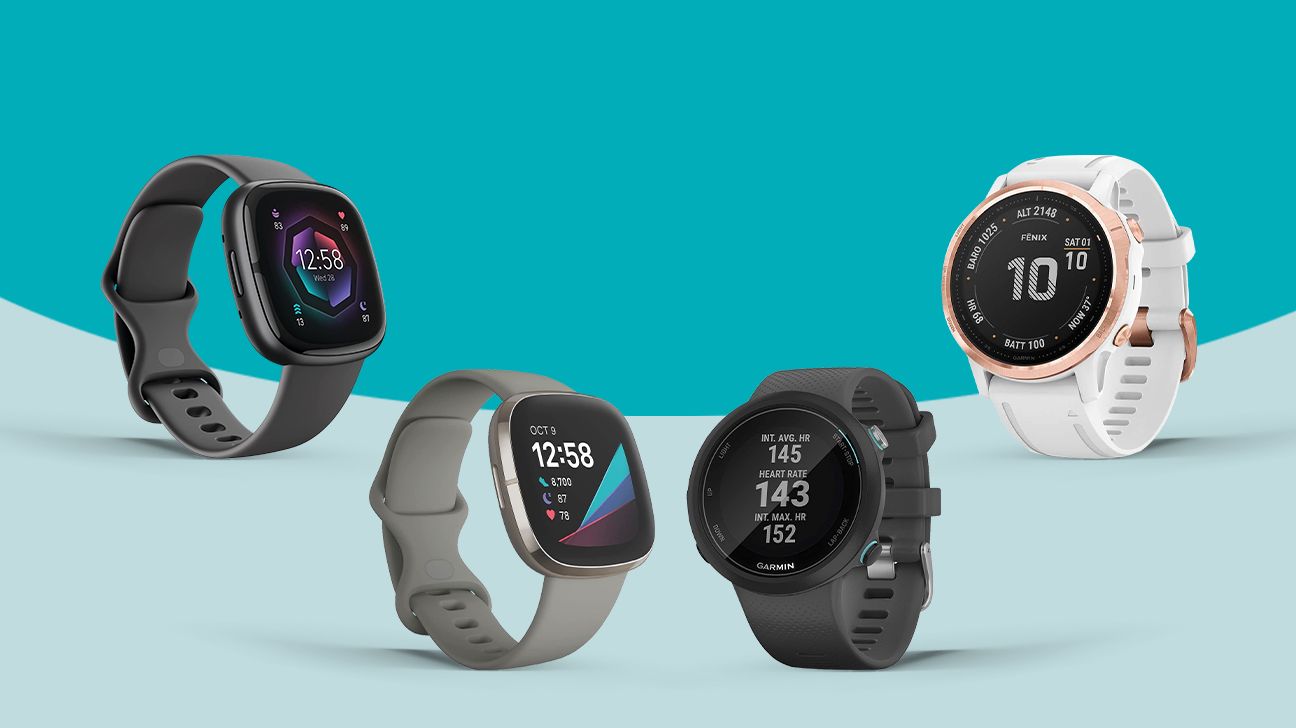The image features a product display of four smartwatches against a white background, accented with a light blue gradient at the top. Each watch has unique features and different data displayed on their screens.

On the upper left, there is a dark gray smartwatch with a rounded square face displaying the time "12:58" and various health metrics, including steps and heart rate, with symbols such as a heart and a moon.

Directly below it sits a slightly lighter gray smartwatch, also with a rounded square face, displaying the same time "12:58".

To the right of these two, the upper middle watch has a black circular face with a dark gray band. This watch shows detailed heart rate statistics: a current rate of "143", an average rate of "145", and a maximum rate of "152".

On the far right, a white smartwatch with a circular face, detailed in rose gold, features the number "10" prominently, with the date "Saturday 01".

Together, the smartwatches present an array of timekeeping and health tracking functions, displayed on sleek, modern digital interfaces with black screens and white fonts.